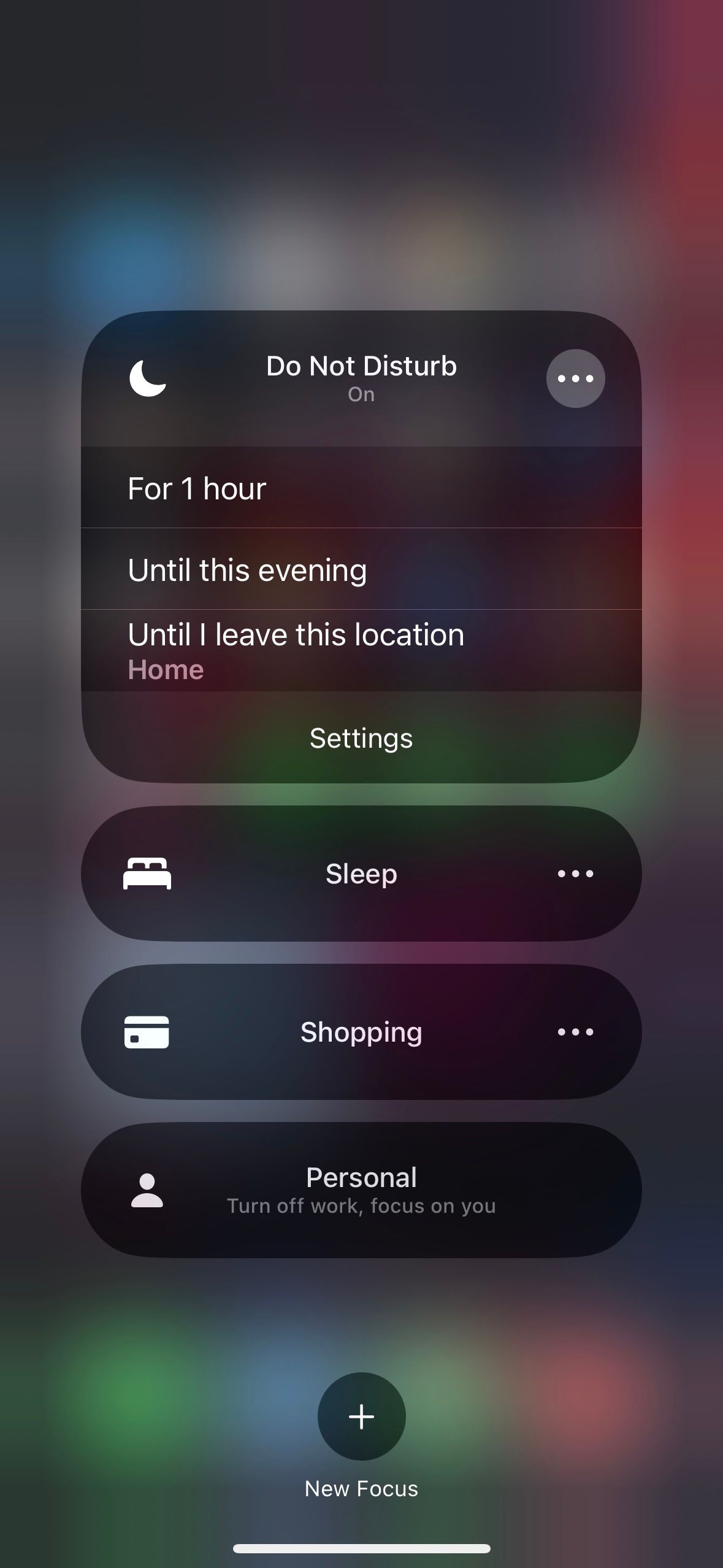Capturing a screenshot of an Apple iOS device displaying the "Focus" settings menu, the background is artistically blurred to emphasize the foreground elements. The interface includes four distinct focus settings, each represented as a bubble with its own unique icon and options.

At the top center, the "Do Not Disturb" bubble is highlighted with a crescent moon icon on the left and a three-dot ellipsis on the right, indicating additional settings. The "Do Not Disturb" is currently activated and offers three customizable options: "For 1 hour," "Until this evening," and "Until I leave this location called Home." The last option directs to "Settings" for further adjustments.

The second bubble, labeled "Sleep," features a bed icon on the left and another three-dot ellipsis on the right for more settings. The third bubble, "Shopping," has a credit card icon to its left and an ellipsis to its right, similarly indicating additional options.

The final focus setting, titled "Personal," encourages the user to "Turn Off Work, Focus on You" and is marked with a silhouette of a person icon on its left. Below these bubbles, at the bottom of the screenshot, there's a circular button with a plus sign labeled "New Focus," enabling the user to create a new custom focus setting.